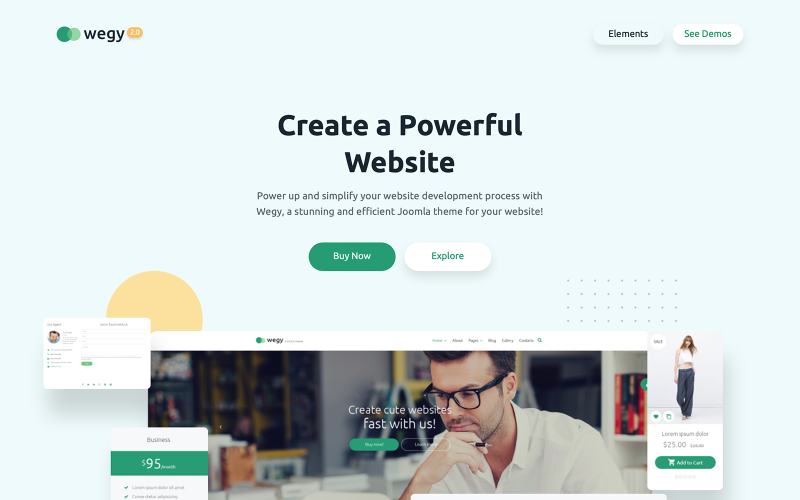The image is a screenshot from a desktop computer, displaying a web page with a background that features a very pastel shade of blue, almost white in color. In the upper-left corner, there is a logo consisting of two intersecting green circles, with the brand name "Wiggy" written in black to the right of the circles. Just above the main content area, towards the upper left side, are two buttons: one labeled "Elements" in black, and another labeled "C Demos" in green.

The main body of the webpage prominently features the phrase "Create a Powerful Website" in black text. Directly below this headline, smaller text reads: "Power up and simplify your website development process with Wiggy. A stunning and efficient Joomla theme for your website."

Towards the lower section of the page, there are two buttons positioned side by side. The button on the left is green with white text that says "Buy Now." The button on the right is white with green text that says "Accept."